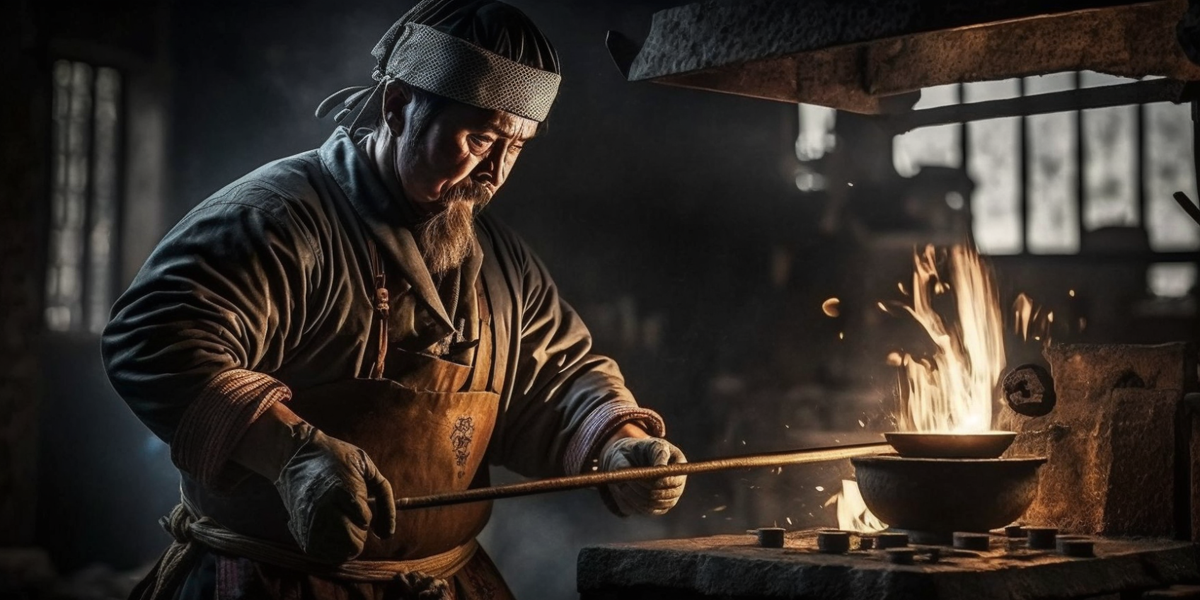In this highly detailed digital illustration, we see an aged Asian artisan, possibly a blacksmith, working meticulously in a dimly-lit workshop. He is wearing a gray headband that holds back his long hair, a brown apron adorned with Asian writing, and heavy leather gloves for protection. His facial features include a mustache and a goatee, with his face illuminated by the intense glow of flames directly in front of him. The artisan holds a long rod with a bowl at the end, which is positioned over another bowl containing heating elements, producing fierce flames and sparks. The room, bathed in shades of brown, has white windows in the background that allow some light to filter in, contrasting with the darkness of the workshop. This captivating scene captures the artisan's focused expression as he engages in the traditional craft of metalworking, with every detail emphasizing the age-old skill and the fiery heart of his trade.